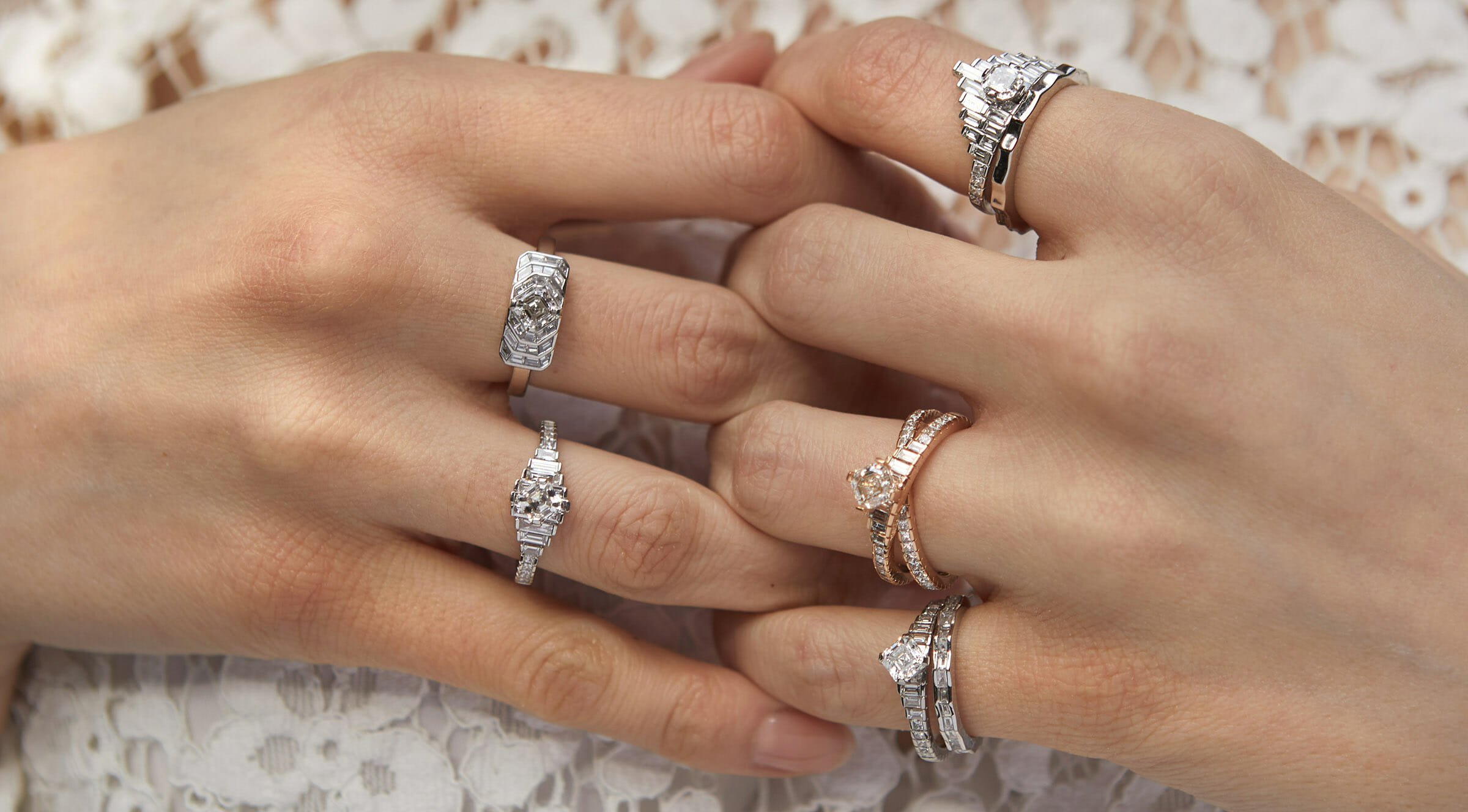This image features a close-up of a young woman's intertwined hands adorned with an array of distinctive rings. Her smooth fingers are elegantly folded together, showcasing five intricate rings on each hand. On her right hand, she wears a silver ring embellished with a diamond on her middle finger and another ornate silver ring with a rectangular piece on her ring finger. Her left hand displays rings on her index finger, ring finger, and small finger, with multiple rings stacked on both her index and pinky fingers, including designs that appear almost like a pipe organ and a band featuring a square inset. The rings exhibit an art deco style with square and diamond shapes, suggesting a non-traditional, possibly wedding-related collection. The background reveals the texture of an off-white, floral lace dress with visible skin through its delicate holes, adding a subtle, yet elegant touch. The lighting casts evenly on her hands, emphasizing the details of the rings and the lace fabric.